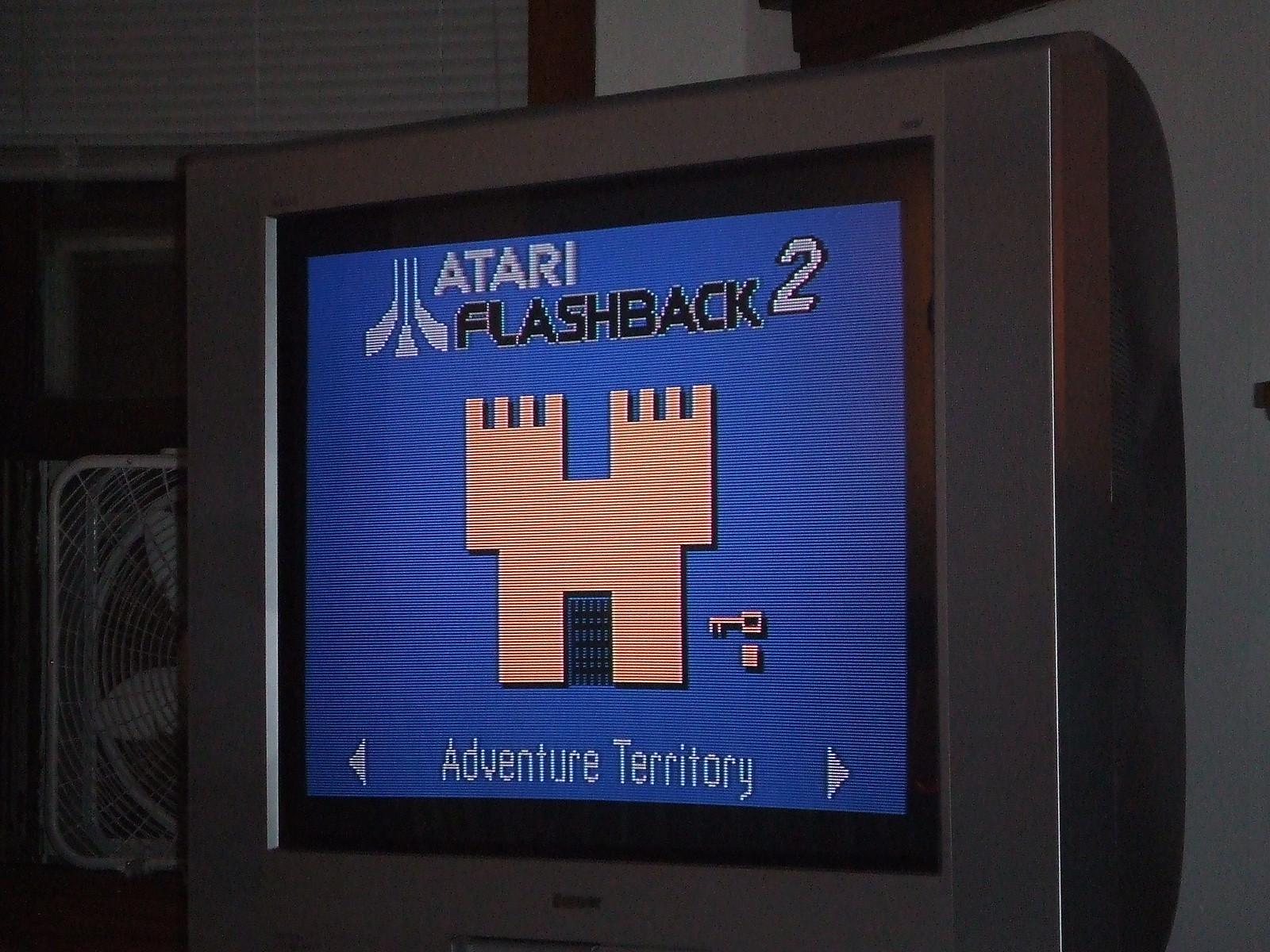This photograph captures a modern individual engaging with an Atari Flashback 2 console on a notably large CRT television, hinting at a nostalgic revival rather than a snapshot from the era when original Atari consoles were prevalent. The screen prominently features the words "Adventure Territory" at the bottom, flanked by white directional arrows pointing left and right. At the top left is the recognizable Atari logo. A simplistic, somewhat crude depiction of a castle with a black gate and a key with a small square beneath it adorn the screen, characteristic of classic Atari graphics.

In the background, a window with white blinds, drawn halfway down, is open, allowing light to filter through. A window fan is positioned within the open window, although it appears to be turned off. Above the TV hangs a wooden shelf against a white wall, adding to the room's casual and lived-in feel. The large CRT TV, likely ranging between 20 to over 30 inches, seems out of place for the Atari era but is utilized here to enhance the visual quality of the retro gaming experience. The entire setup underscores the practice of using CRT televisions to play vintage games, as these displays are better suited to the output of older consoles.